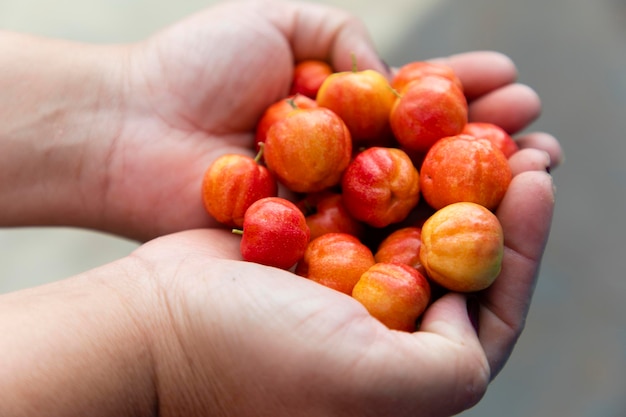The photograph features two bare-skinned hands extended from the left side of the image, with wrists partially visible against a grayish-cream background. The hands are cupped together, forming a bowl-like shape and holding a collection of small, round fruits. These fruits, which vary in color from red to orange, yellow, and hints of green, resemble crab apples or possibly some kind of berry. The fruits are numerous, with estimates ranging from about 15 to 20 or more, displaying different stages of ripeness as indicated by their varied hues. Some of the fruits have tiny stems protruding from the top, and they appear hard and ridged in texture. The image is realistic and solely focused on the hands and the fruits, without any additional text or elements.